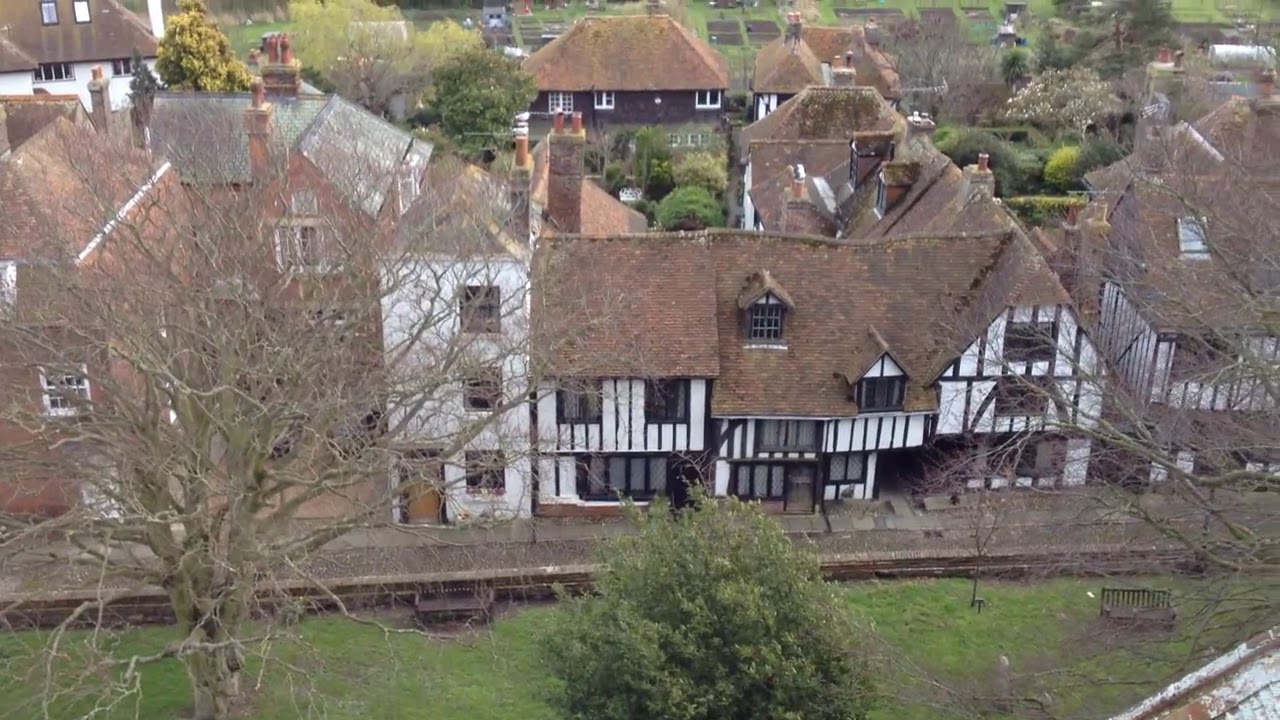This aerial photograph, taken from a downward perspective, showcases a diverse array of tan, brown, white, and cream-colored houses and buildings clustered in an urban neighborhood. The structures predominantly feature slanted brown roofs. Central to the image is a prominent Tudor-style house distinguished by its white exterior with vertical brown patterning, two dormer windows, and a large gable on the right. This building is flanked by a three-story white building on one side and a two-story brick building on the other.

In the foreground, a grassy lawn area is peppered with bushes and trees, including a notable large, leafless tree on the left side. The setting is outdoors, bathed in the light of midday, with various sidewalks and pathways visible among the residential buildings. The photograph captures shades of green, brown, white, red, orange, and gray. In the background, a mixture of buildings can be seen interspersed with a variety of trees, adding depth and context to the urban landscape. The image epitomizes photographic realism through the clear, detailed view afforded by the drone, highlighting the intricate interplay between architecture and nature.